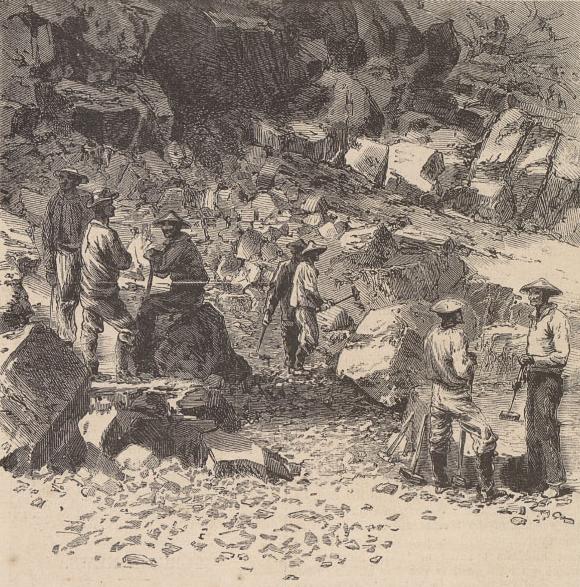This vertically-oriented sepia-toned sketch depicts a group of old-fashioned, possibly Asian miners working on the side of a rocky mountainside. The image, rendered in black and white, displays a rugged terrain with boulders and rock fragments scattered across the ground. Various workers are gathered in small groups, equipped with tools such as chisels and mallets. On the right side, two men—clad in long-sleeve shirts, pants, and one in high boots—are engaged in conversation, with the taller man holding a tool. In the central area, more miners can be seen wearing distinctive triangular hats, strikingly reminiscent of pointed sun hats. One central figure is actively chiseling a large boulder. To the left, three men—one seated on a rock and two standing—appear to be discussing their work. The rocky landscape extends upwards, forming a rugged wall, and the scene vividly captures the gritty essence of the manual labor involved in mining.